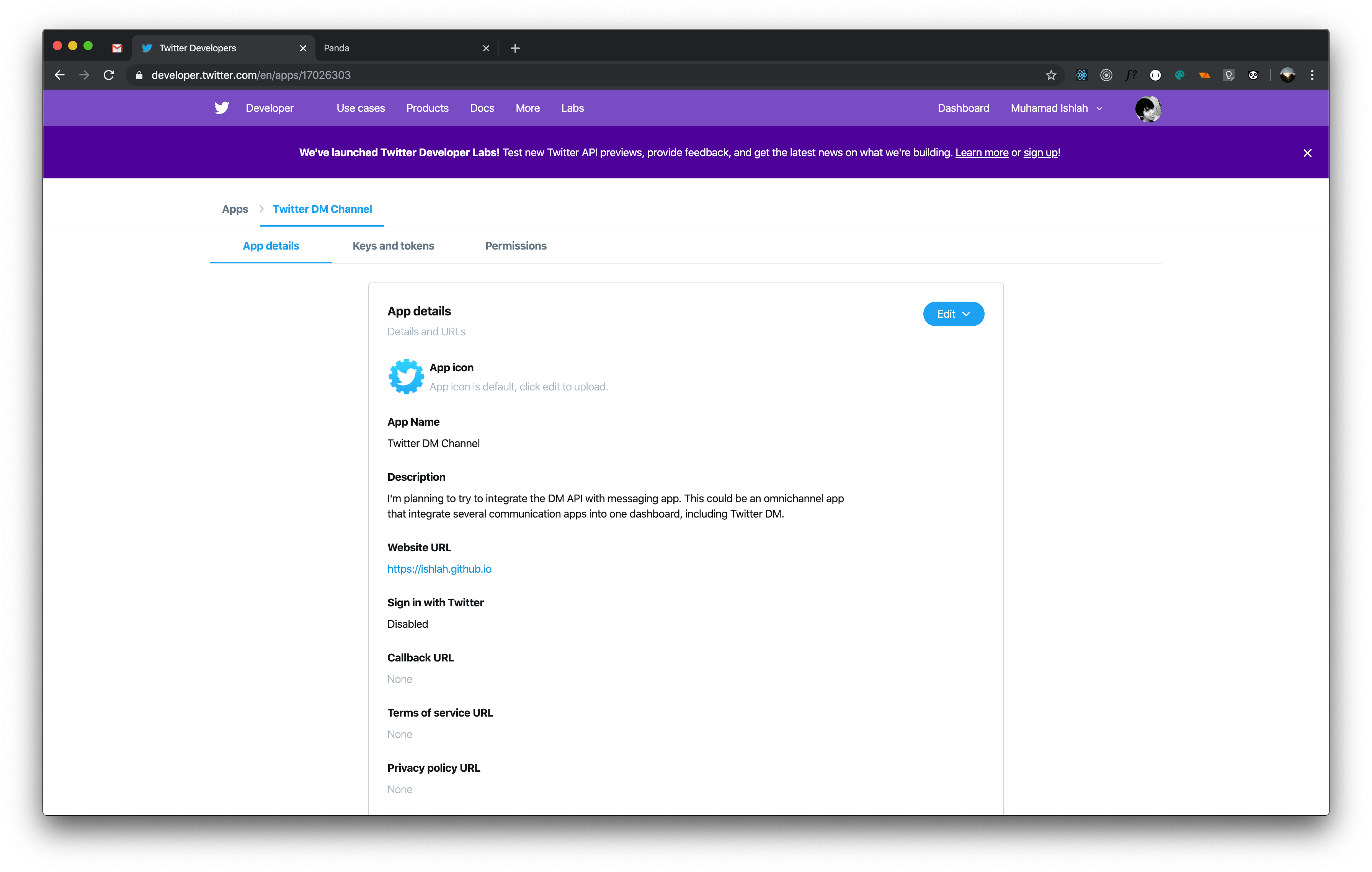A screenshot of a developer's Twitter dashboard on a Mac. The top-left corner features the characteristic Mac control buttons in red, yellow, and green. The browser has multiple tabs open, with the primary focus on the "Twitter Developers" tab. Next to it is another tab labeled "Panda".

The URL displayed in the address bar is "developer.twitter.com/apps/..." indicating a specific app page. Below the URL, the website's navigation bar is visible, showcasing options such as Home, Use Cases, Products, Docs, More, Labs, and a dashboard link. To the far right of the navigation bar, there's a profile section with the name "Muhammad Aishla" and a profile picture dropdown.

A prominent banner announces the launch of Twitter Developer Lateral Tests, offering new Twitter API previews and inviting users to learn more or sign up via clickable links.

The main content area displays the "Apps" section, highlighting the "Twitter DM Channel". This is further divided into three tabs: "App Details," "Keys and Tokens," and "Permissions," with the "App Details" tab currently active and highlighted in blue. Within the "App Details" tab, there's an edit button in blue.

Details of the Twitter app are listed next, starting with the app icon, followed by "App Name: Twitter DM Channel". A detailed description states: "I'm planning to try to integrate the DM API with messaging apps. Could be an omni-channel app that integrates several communication apps into one database, including a Twitter DM." Below this, there are various URLs: Website URL (clickable link), Sign in with Twitter (disabled), Callback URL (None), Terms of Service URL (None), and Privacy URL (None).